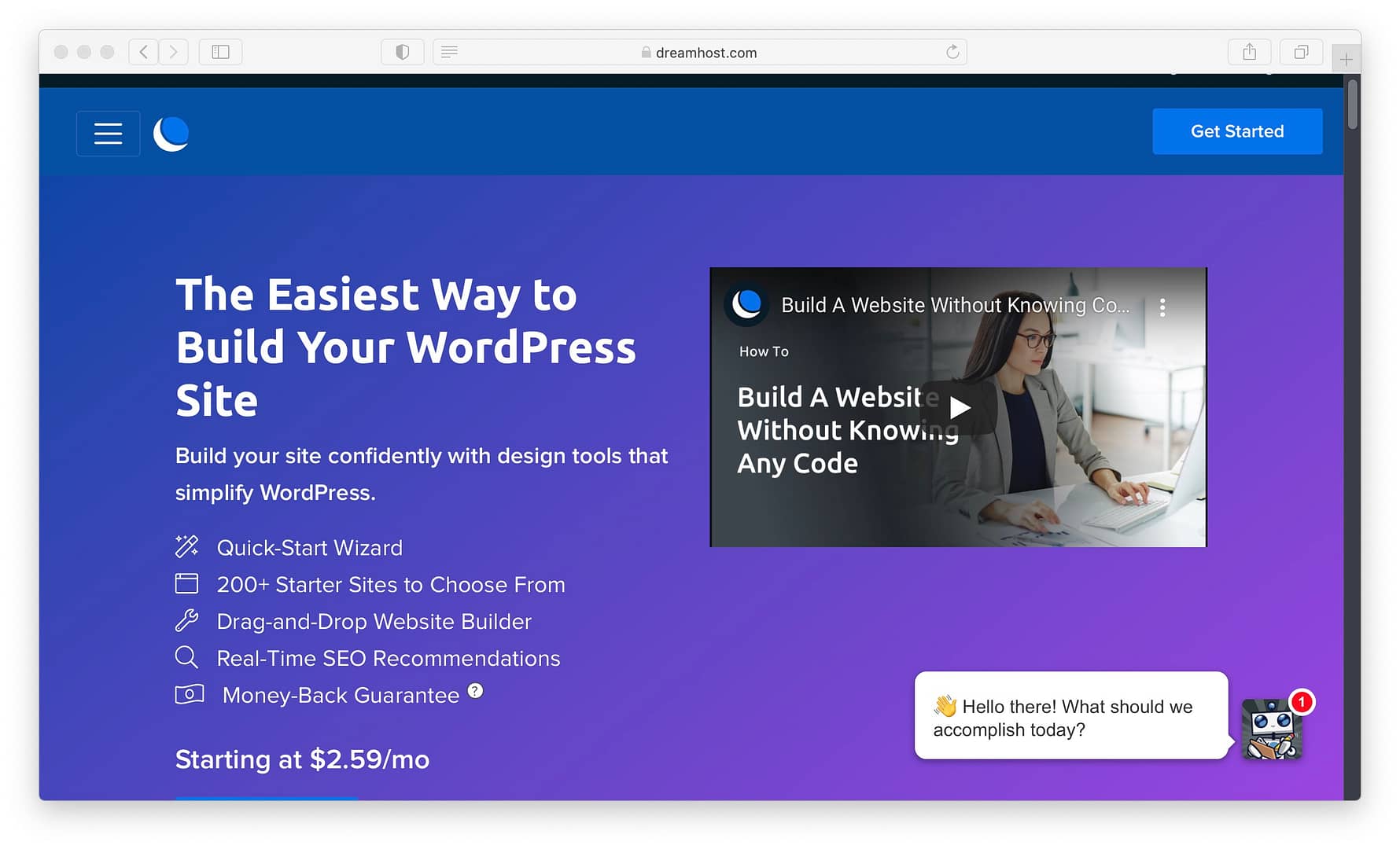The DreamHost.com website features a sleek bluish-purple background aimed at simplifying the WordPress site-building process. The headline reads, "The Easiest Way to Build Your WordPress Site," emphasizing confidence through user-friendly design tools. Key features listed include a Quick Start Wizard, 200 starter sites, a drag-and-drop website builder, real-time SEO recommendations, and a money-back guarantee starting at $2.59 per month. 

On the right side of the page, there is an embedded YouTube video cover photo showing a woman with glasses and a gray blazer working on a laptop in an office setting. The video, titled "How to Build a Website Without Knowing Code," can be played directly on the site. Additionally, a chatbot icon, illustrated as a cute metallic robot, is located at the bottom right corner with the prompt, "Hello there, what should we accomplish today?"

A prominent "Get Started" button in blue is positioned at the top right, while a crescent moon icon on the top left possibly toggles between light and dark modes. A nearby menu button likely reveals a left pane with additional navigation options when clicked.